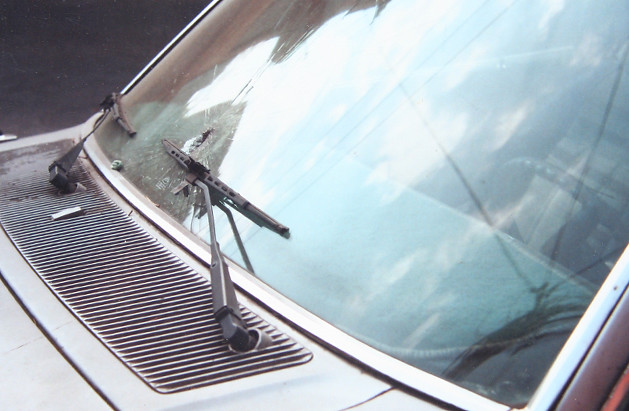This photo captures a partial view of an older car, focusing on the hood and windshield. The vehicle's color appears to be silver or champagne. Prominently featured are the windshield wipers, nearly in the down position, connected to an air vent or grate that stretches across the top of the hood. The windshield itself shows reflections of clouds, blue sky, and sunlight, with some parts also reflecting buildings and possible telephone wires.

A significant detail is the damage to the windshield. On the passenger side, there is a large, conspicuous hole surrounded by networked cracks, characteristic of a tempered glass shattering. Near the damaged area, a rock can be seen laid underneath one of the wiper blades, suggesting it may have caused the damage. The windshield wipers, along with the glimpse of the car’s interior, including the steering wheel, seats, and dashboard, add to the detail of the scene, suggesting a moment captured post-impact, potentially from an object falling onto the windshield rather than a collision.